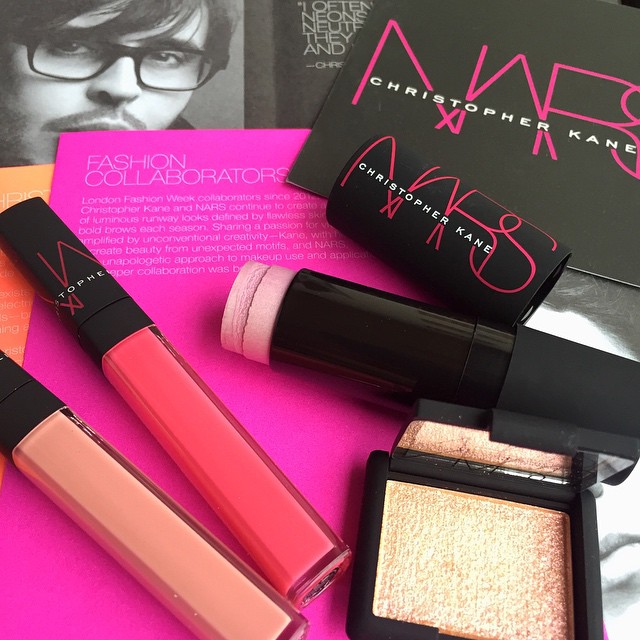This photograph appears to be a social media advertisement, possibly aimed at platforms like Instagram or Facebook. It features a display of makeup products arranged over a couple of pamphlets. The backdrop primarily includes a pink pamphlet with white text reading "Fashion Collaborators," and a mention of "London Fashion Week Collaborators since 2012." Part of the text is obscured, but it highlights a collaboration between Christopher Kane and NARS.

The makeup items include a gold-looking blush, an orange tube with a black cap, and two cream-colored glass tubes. Each item is marked with the names Christopher Kane and NARS, signifying their collaboration. There also appears to be a mirror in the bottom right, complementing the makeup products. In the background, there is a black-and-white photograph of a man with a mustache, long dark hair partially covering his eyes, and dark-framed glasses. 

Overall, the photograph is designed to highlight these makeup products and their association with renowned fashion collaborators, set against an aesthetically structured background that merges both black-and-white and colored elements.